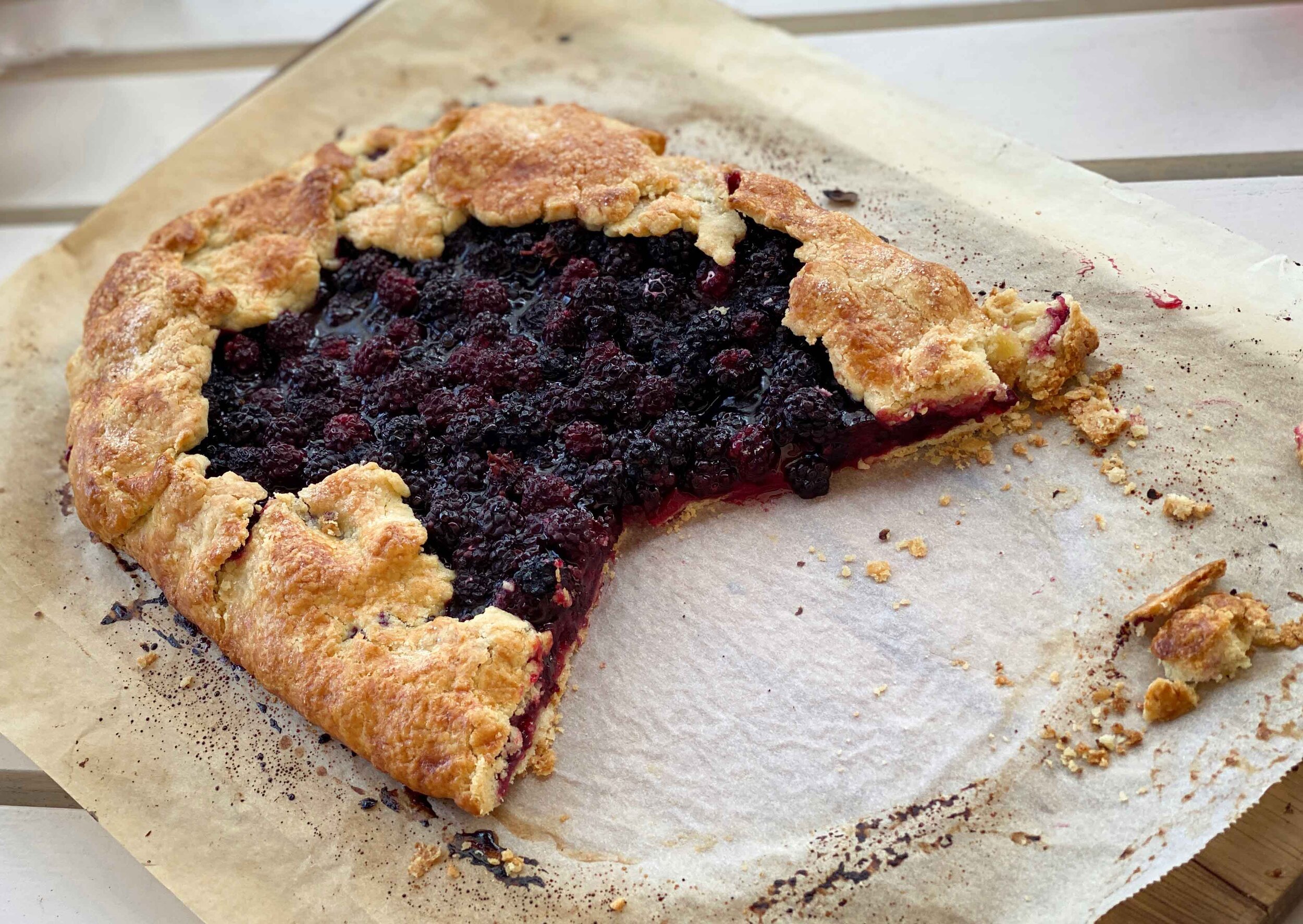The color photograph captures a picturesque rustic blackberry galette, or tart, resting on a parchment paper lined baking sheet. The galette has an oblong shape with irregular, jagged edges of the crust, simply folded over to create a rough, approximately one to two-inch border around the blackberry filling. The blackberry filling is dark, juicy, and glistening with rich hues of black, purple, and hints of pink. A substantial wedge has already been cut out, revealing clean, diagonal slices and a few scattered crumbs. In the background, white slats of a picnic table provide a contrasting backdrop, heightening the rustic appeal of this delightful dessert.